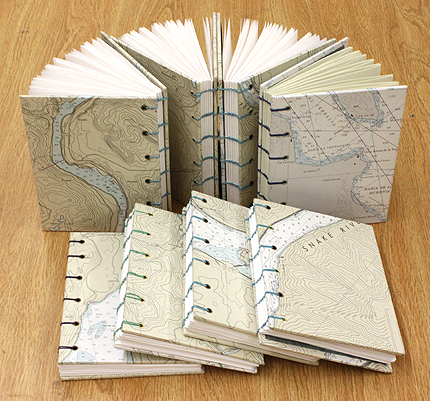The image features a visually striking arrangement of eight books displayed on a light wooden table. In the foreground, four books are laid horizontally in a cascading fashion, each resting on the edge of the one beneath it, revealing only the left half of each book except the one on the right. These covers are a light pinkish-brown with intricate designs resembling maps, showcasing white streams lined with black polka dots. Binding these books is a teal string threaded through the spine. 

Behind this horizontal stack, four additional books stand upright, fanned out to create a semicircle with approximately 45-degree angles between each. These standing books share the same topographical map-like covers, emphasizing geographic features such as elevation lines and rivers. This symmetrical yet dynamic arrangement showcases the books in a way that highlights their unique designs and delicate bindings.